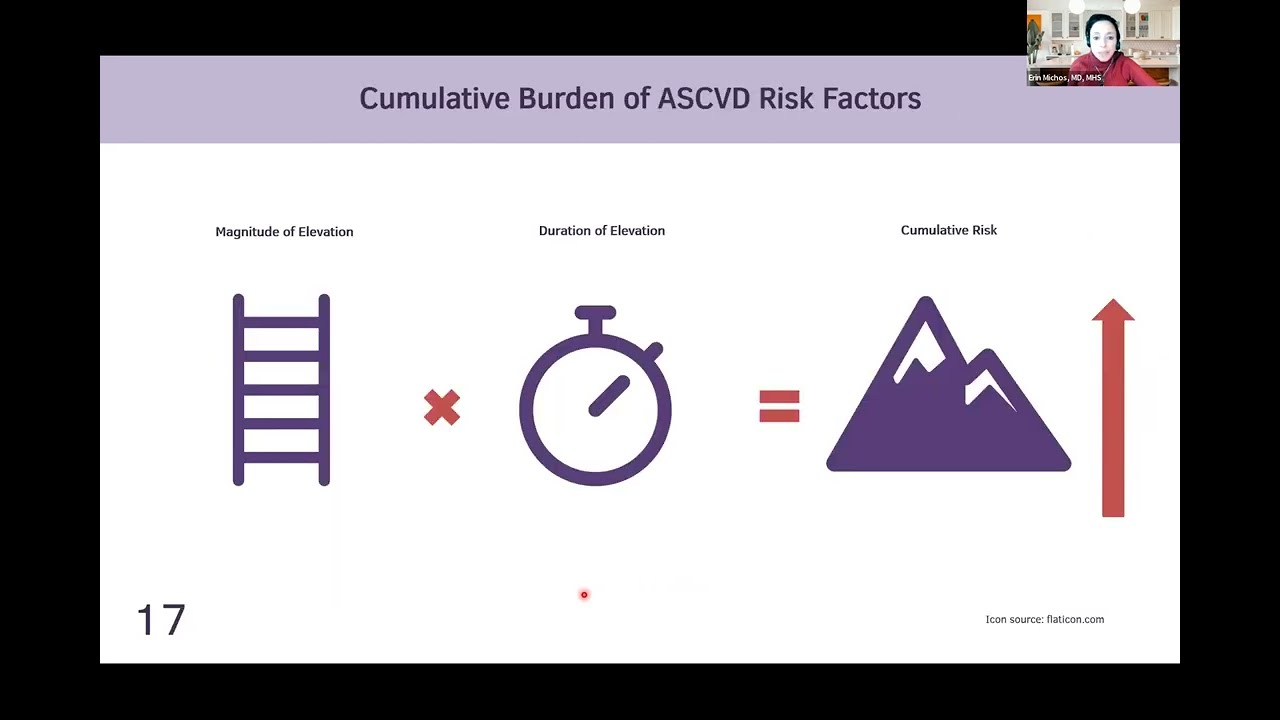The image is a detailed screen capture, likely from a PowerPoint presentation, featuring slide 17. The slide has a half-inch thick black border. In the top right corner, there is a small thumbnail of a webcam capture showing a woman with black hair and glasses, wearing a red turtleneck, sitting in what appears to be a kitchen area as she looks at her computer screen. Below the webcam thumbnail, a light purple banner displays the text "Cumulative Burden of ASCVD Risk Factors" in black font. Central to the slide are three graphical elements: a ladder labeled "Magnitude of Elevation," a clock labeled "Duration of Elevation," and a mountain icon beside an upward-pointing arrow labeled "Cumulative Risk." These elements are shown with mathematical signs, including a multiplication symbol between the ladder and the clock, and an equal sign leading to the mountain icon with the arrow. Additionally, the bottom left of the slide features the number 17, and the bottom right corner includes the text "Icon Source, FlatIcon.com."